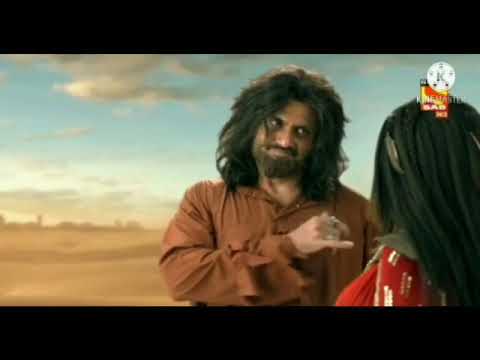In a desert setting with a sandy expanse and a slightly cloudy sky that transitions from brownish near the horizon to blue above, a man with long, scruffy black hair and a thick beard gazes down at a woman who is shorter than him. The man, dressed in a puffy brown garment reminiscent of pirate attire, adorned with large sleeves and multiple silver rings on his fingers, uses his pinky finger to point at the woman. His hair reaches his shoulders, matching his unkempt look. The woman, visible from the back and side profile, has long black hair and wears a red blouse detailed with gold rectangular accents on the shoulders. In the upper right corner of the image, there's a white logo featuring the letter "K" inside a circle, placed over a small red rectangle. The backdrop features distant cliffs under a double moon, lending an otherworldly feel to the scene. The image is framed by thin black borders at the top and bottom, giving it a polished look.